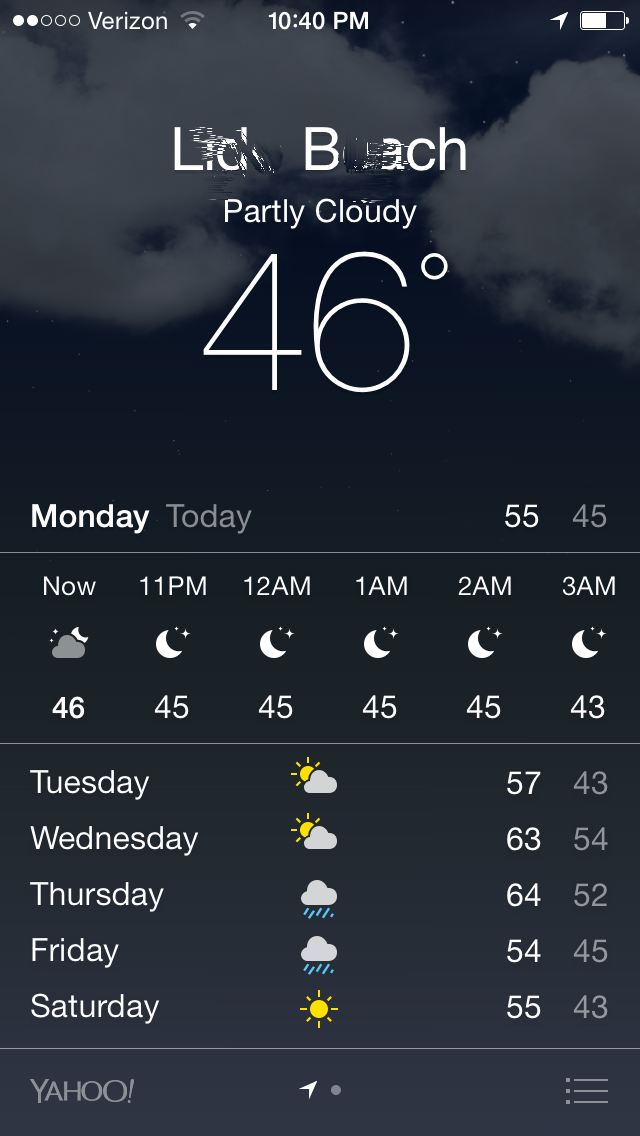The image is a detailed screenshot taken in portrait mode from a cell phone, displaying a weather forecast page. The background features a very dark blue sky with scattered white clouds. 

In the upper left corner, two out of five signal strength circles and the "Verizon" carrier name are visible. At the top center, the time is displayed as 10:40 PM, while the upper right corner shows the battery icon, which appears to be approximately 50% or more full.

An address is listed but has been crossed out for privacy. It appears to be either Lido Beach or Lick Beach, California. Below the address, the current weather condition is described as "Partly Cloudy" with a temperature of 46 degrees Fahrenheit.

The forecast is presented in the form of a table. The first row displays "Monday" (highlighted) and "Today," with a high of 55 degrees and a low of 45 degrees. A line separates this from the hourly forecast, which lists the hours from 11 PM to 3 AM. Next to each hour, an icon representing the moon's phase is shown, with corresponding temperatures: 46, 45, 45, 45, and 43 degrees Fahrenheit, indicating a trend towards cooler temperatures.

A second line separates the daily forecast for the upcoming days: Tuesday, Wednesday, Thursday, Friday, and Saturday. Icons next to each day represent the expected weather conditions (partly cloudy, rainy, etc.), with Saturday showing a sunny forecast. Temperature ranges for these days are provided, with Saturday expected to be between 55 and 43 degrees Fahrenheit.